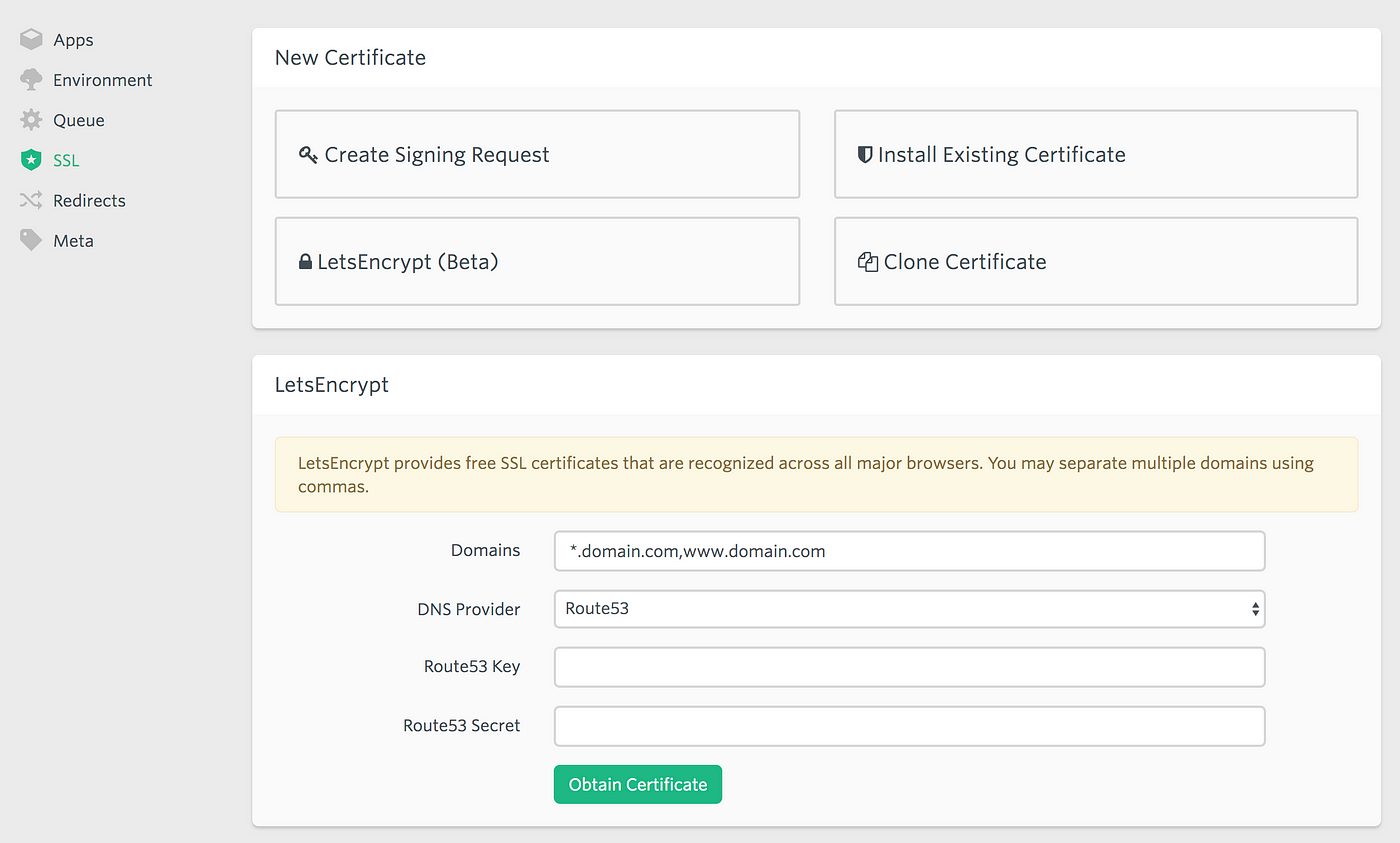The image depicts a screenshot of an SSL certificate management interface, possibly from the program Let's Encrypt. The page features a light gray background and a vertical menu on the left side with options such as Apps, Environment, Queue, SSL, Redirects, and Meta. The SSL section is highlighted in green, indicated by both green text and a green icon. 

The main content area displays various functions related to SSL certificates. These options include creating signing requests, installing existing certificates, cloning certificates, and a beta feature for Let's Encrypt. At the bottom of the page, it is mentioned that Let's Encrypt provides SSL certificates recognized by all browsers. 

To obtain a certificate, users are prompted to enter their domain name, DNS provider, Route 53 key, and Route 53 secret. This ensures the website's security through encrypted connections, thereby protecting data and interactions for site visitors.